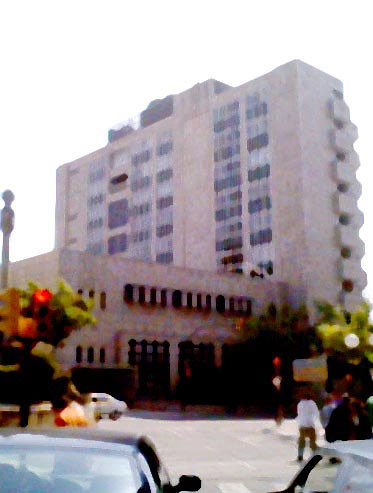The photograph depicts a multi-story building that appears very out of focus and blurry, giving everything a distorted, almost pixelated look. The building is in two sections: a smaller, square-shaped portion on the left and a taller, rectangular portion on the right, both made of a light tan or stone-like material. The left section features three large doorways at the front, while the taller right section has multiple windows and an open-air staircase with a stone railing. The blurred white sky indicates that the photo was taken during the day.

In the foreground, there is a busy street with various elements. On the left side of the image, partially obscured, is the hood of a black car, while on the right side, the side and roof of a gray car are visible. A human figure, dressed in dark pants and a light-colored shirt, is walking near the center-right of the image. Amid the scene are plants and some trees with indistinguishable green foliage flanking the building. There are also traffic lights and street poles scattered throughout the scene, but no discernible text or signage. The overall setting is of an urban street with the building in the background and various elements adding to the busy, bustling atmosphere.